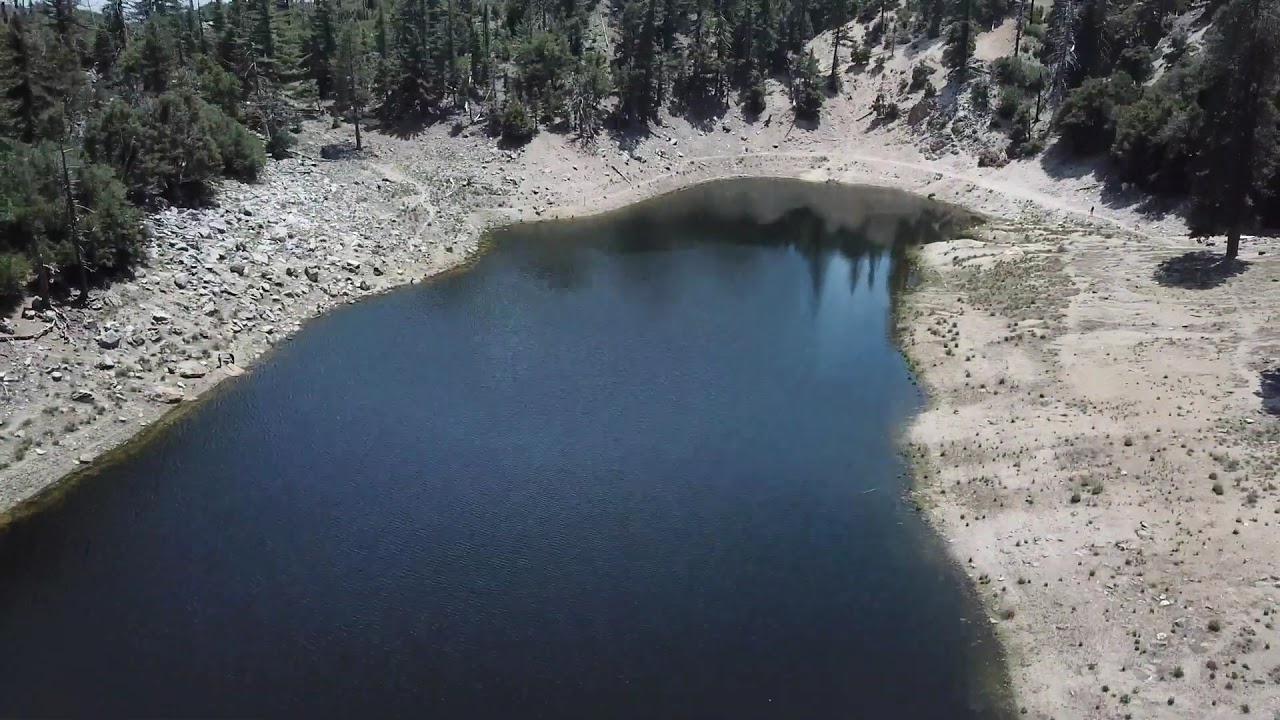This detailed aerial photograph taken during the daytime showcases a mountain lake surrounded by nature. Occupying the entire center of the image, the lake's distinct dark blue water, almost black in some areas, reflects the surrounding trees. Shaped somewhat like the Oogie Boogie character from "The Nightmare Before Christmas," the lake's wide bottom narrows as it extends upward, with two wider outlets before tapering to a curved point. The shore is lined with light tan to almost white sand interspersed with stones, contrasting the dark waters. Small green bushes and shrubs dot the shoreline, with a small visible path at the top end. Behind this sandy perimeter, tall evergreen pine trees ascend steeply, marking the edge of the mountain. The right side of the shore is particularly sandy and cream-colored, while distant mountain peaks can be subtly seen through the trees on the left, hinting at the path's direction.